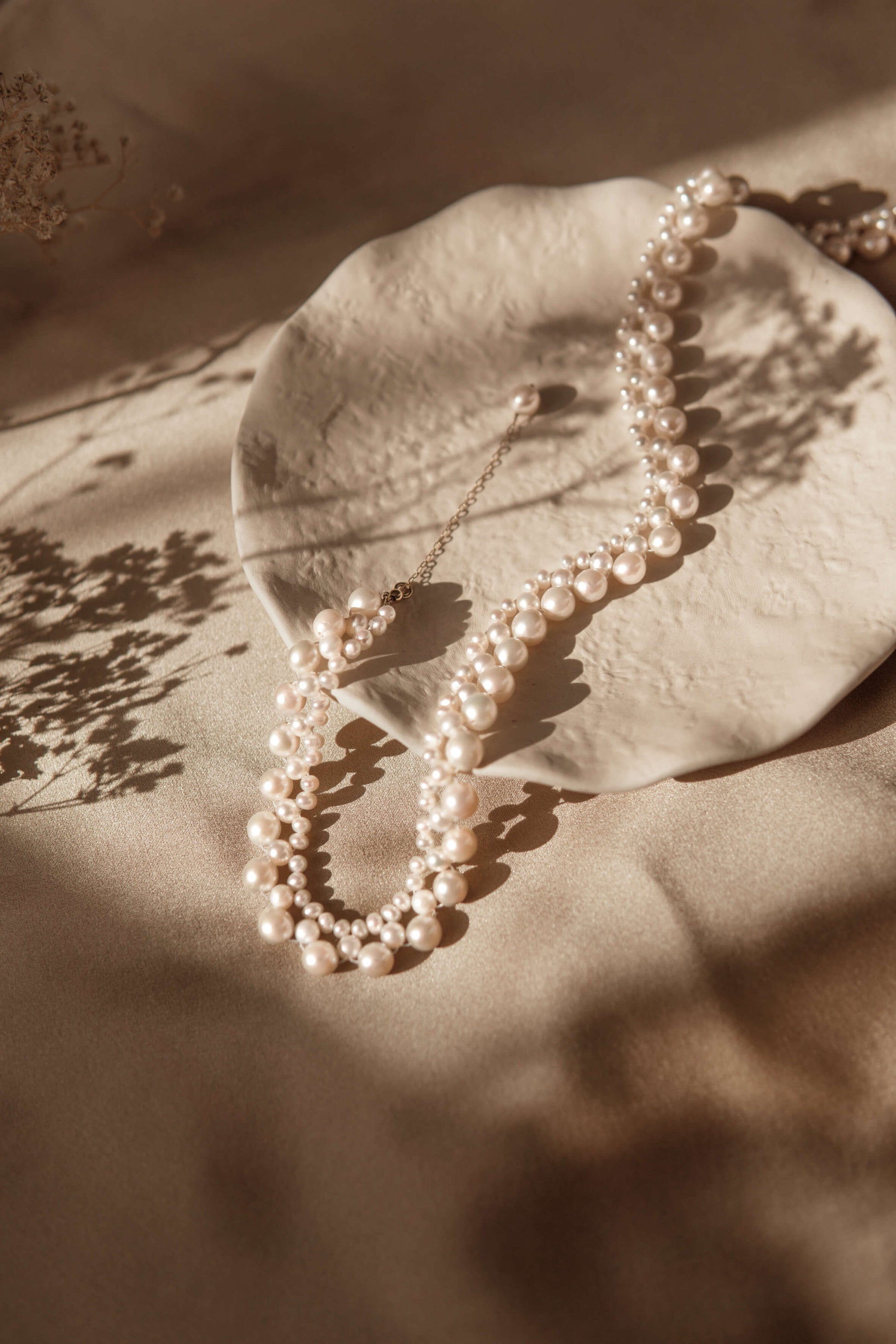The image features an elegant and shiny pearl necklace composed of various sizes of white pearls, with smaller pearls interspersed between larger ones, giving it a luxurious and expensive appearance. The necklace, which appears to be unclasped, is artfully draped over an irregularly shaped, wavy dish with a shell-like texture, showcasing its bumpy and rough surface which is off-white in color. The dish sits atop a light beige sheet that has a sandy texture, partially covering the necklace. The scene is made more captivating by dramatic lighting, casting shadows from nearby plant leaves over the pearls and the dish, giving the photograph a stylized and alluring appearance, as if it were an advertisement for the fine jewelry.